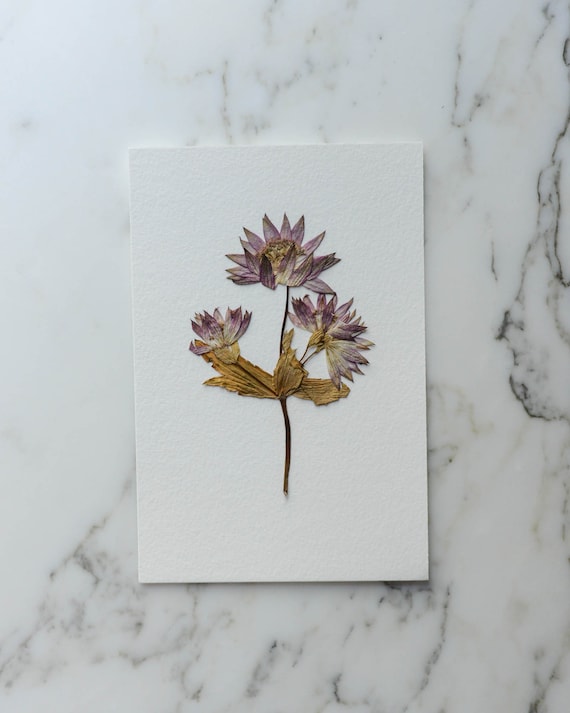The photograph showcases a detailed and vibrant composition. At its foundation, the background is a stunning white marble slab with swirling patterns of black and gray, accentuating the sleek and polished texture. Centered on this elegant marble lies a piece of white cardstock, distinctly shaped like a triangle, providing a clean and contrasting canvas. Affixed to the cardstock is a meticulously pressed, dried flower. The flower features a dark, slender stem, and its spiked petals display a spectrum of colors, primarily purple with hints of gray. The flower blossoms radiate outward, resembling the rays of a half-sun, with petals transitioning from purples and pinks to vibrant oranges and yellows, anchored by a brownish-yellow foliage. This harmonious blend of natural elements and geometric precision evokes a sense of preserved beauty, making it reminiscent of an artistic piece suitable for a greeting card or a delicate piece of wall art.